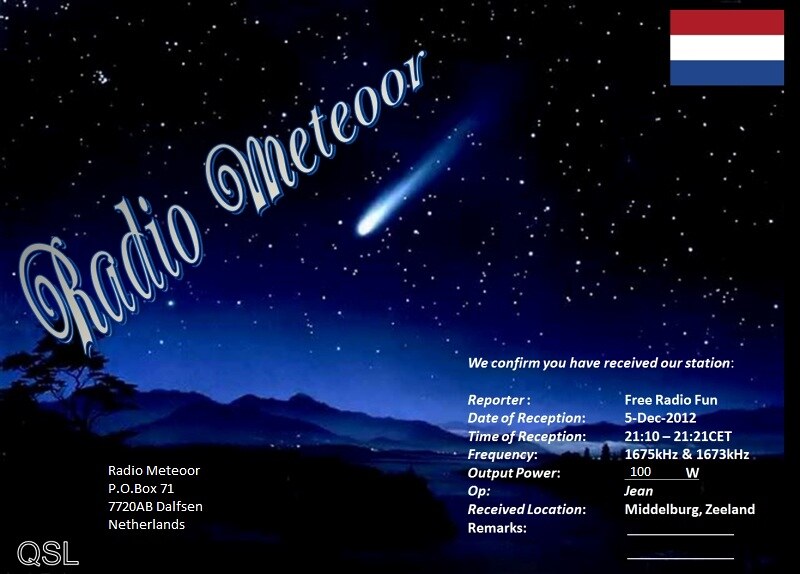The image is a detailed poster for "Radio Meteor" set against a stunning night sky backdrop. The sky is predominantly dark, featuring numerous twinkling stars, with a bright, white meteor streaking across, symbolizing the core theme of the poster. Illuminating the land below in a striking blue hue, the glow from the meteor casts shadows on the hills and trees, adding a mystical touch to the scene. Prominently displayed in white type across the sky is the name "Radio Meteor," accompanied by the text "We confirm you have received our station."

In the upper right-hand corner of the poster, there is a flag with three horizontal stripes: red on top, white in the center, and blue at the bottom, identified as the flag of the Netherlands. The bottom left corner features the logo "QSL" and below it, the detailed mailing address: "Radio Meteor, PO Box 71, 7720AB Debsen, Netherlands."

The bottom right side contains further information, specifying reception details including the date (5 December 2012), time (2110 CET), frequency (1675 kHz and 1673 kHz), output power (100 watts), the operator's name (Gene), and the received location (Middelburg, Zeeland). Remarkably, there are also two blank lines present on the poster, likely for additional notes. The combination of these elements, along with the detailed nighttime setting, makes for a visually appealing and informative poster.